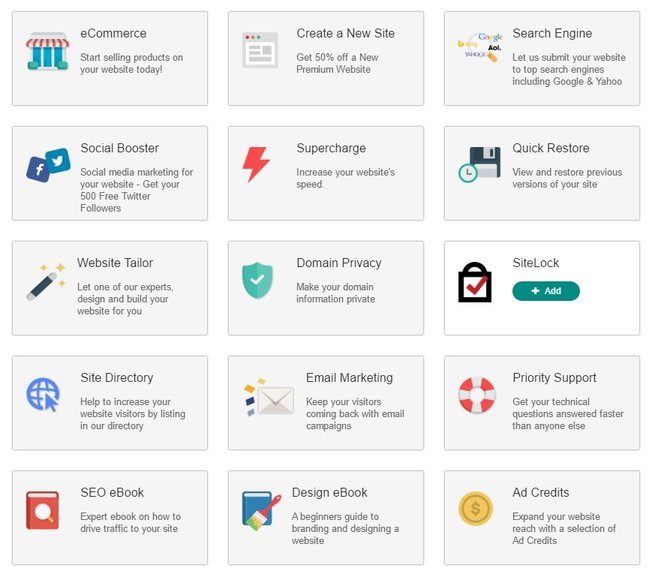The image features a group of rectangles, primarily in gray, each containing various icons and text descriptions. Here is a detailed description of the contents of these rectangles:

1. **E-commerce**: The top-left rectangle showcases an image of a building and the caption "E-commerce" at the top, followed by additional descriptive text.
   
2. **Create a New Site**: To the right, there is an icon resembling a disk embedded with various colored dots, labeled "Create a New Site" with text underneath.
   
3. **Search Engine**: This rectangle displays several indistinct symbols and the label "Search Engine," with further descriptive text below.
   
4. **Social Booster**: Moving back to the left, beneath the initial rectangle, there are Facebook and Twitter icons alongside the label "Social Booster" and supplementary text.
   
5. **Supercharge**: Next, an icon of a red lightning bolt accompanies the label "Supercharge" and additional descriptive words.
   
6. **Quick Restore**: Featuring an icon of a disk with a green-outlined circle and clock hands inside, this one is labeled "Quick Restore" with more text following.
   
7. **Website Tailor**: On the lower-left side, a pencil surrounded by yellow stars indicates the "Website Tailor" option, with subsequent descriptive text.
   
8. **Domain Privacy**: An icon of a shield with a check mark represents "Domain Privacy" alongside more descriptive words.
   
9. **Site Lock**: This is the only rectangle with a white interior and gray outline. It displays a lock with a check mark and is labeled "Site Lock." It also features a greenish button with a plus sign and the word "Add."
   
10. **Site Directory**: Back on the left side, an icon resembling a globe with an arrow is captioned "Site Directory," with more text below.
   
11. **Email Marketing**: This rectangle includes an envelope icon with colored boxes beside it and is labeled "Email Marketing" followed by additional text.
   
12. **Priority Support**: Featuring an icon of a rescue flotation device, this section reads "Priority Support" with further words beneath.
   
13. **CEO Ebook**: An icon of a book with a magnifying glass is labeled "CEO Ebook," followed by more descriptive text.
   
14. **Design Ebook**: A blue rectangle with a white line at the top and a paintbrush with a red handle and green paint represents the "Design Ebook" section, with additional text below.
   
15. **Add Credits**: Lastly, a yellow circle with a gold outline and a dollar sign marks the "Add Credits" section, accompanied by subsequent words.